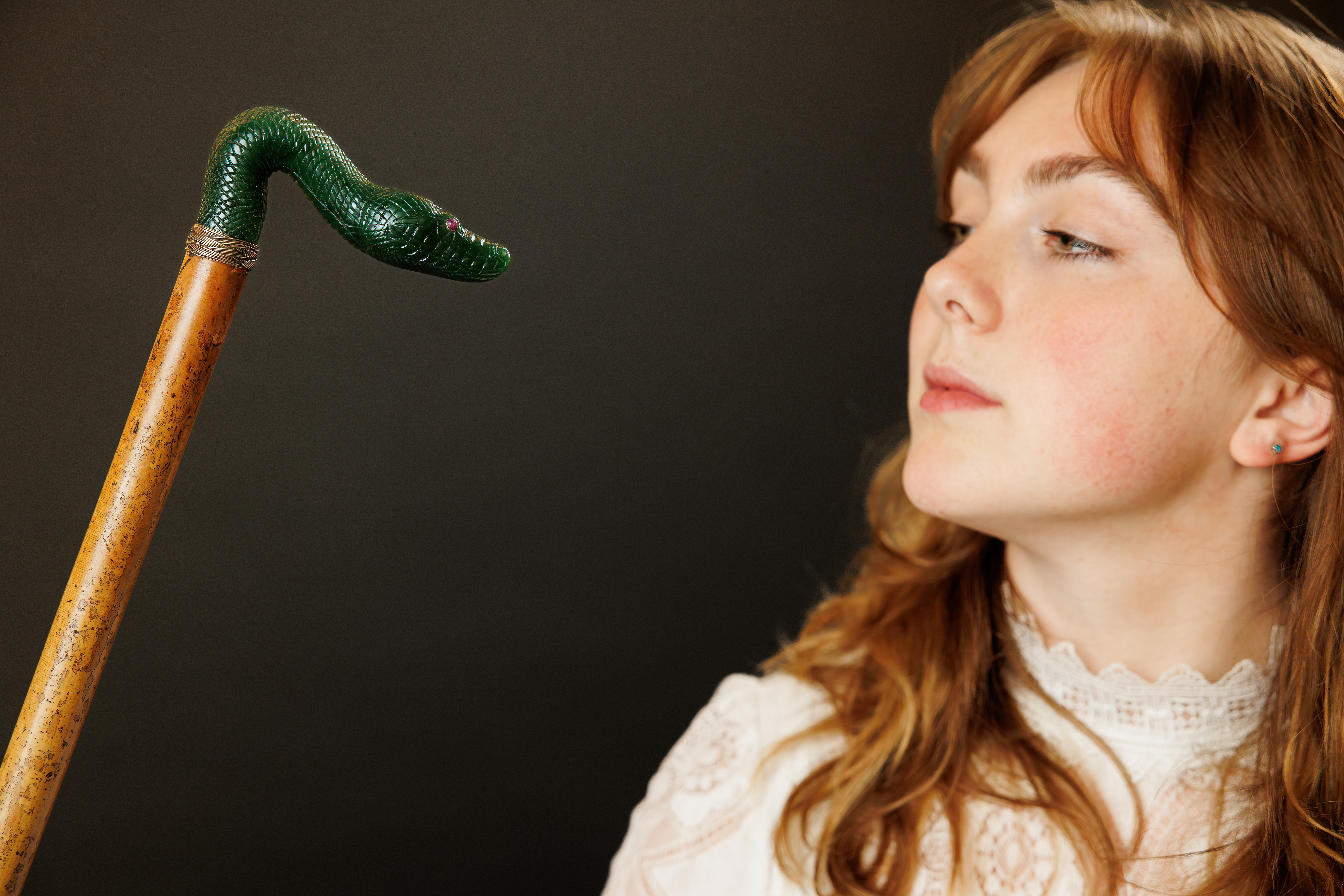In this detailed photograph, a young woman with long reddish-brown hair and thick eyebrows stands on the right, her head slightly tilted back as she gazes down at a cane situated on the left. The cane, made of polished light brown wood with black speckles, extends diagonally upwards from the bottom left. Its handle is intricately designed to resemble a serpent's head and neck, with a sinister black and dark green coloration and red eyes that seem to stare back at the woman. The young woman’s pale face is framed by her loose hair, and she wears a high-collared, intricately laced white top, which adds a vintage charm to her appearance. A small blue earring dangles from her ear, subtly peeking through her hair. The background of the image is a dark, blackish-gray hue, which accentuates the central figures and their focused interaction.